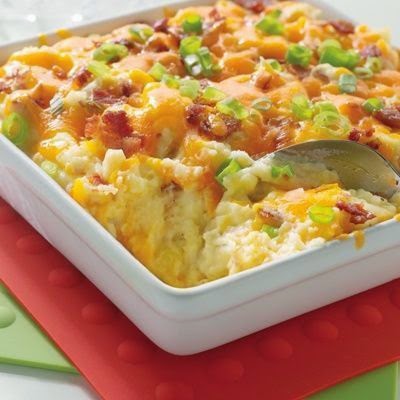The image showcases a close-up of a square white ceramic dish containing a hearty breakfast casserole, prominently positioned on a red silicone mat with a green silicone mat underneath, all resting on a white countertop. The casserole dish, almost filling the entire frame, displays a warm, inviting dish that appears to be a loaded mashed potato casserole or egg-based breakfast bake. The top layer is generously covered with melted cheese, thinly sliced green onions or chives, and what looks like bacon bits or possibly pepperoni slices. A silver spoon, partially visible with its handle cut off, is embedded in the dish with a scoop already taken out, suggesting it’s ready to serve. The vibrant colors and detailed textures of the casserole's ingredients and the distinct trivets beneath create an appealing culinary presentation.